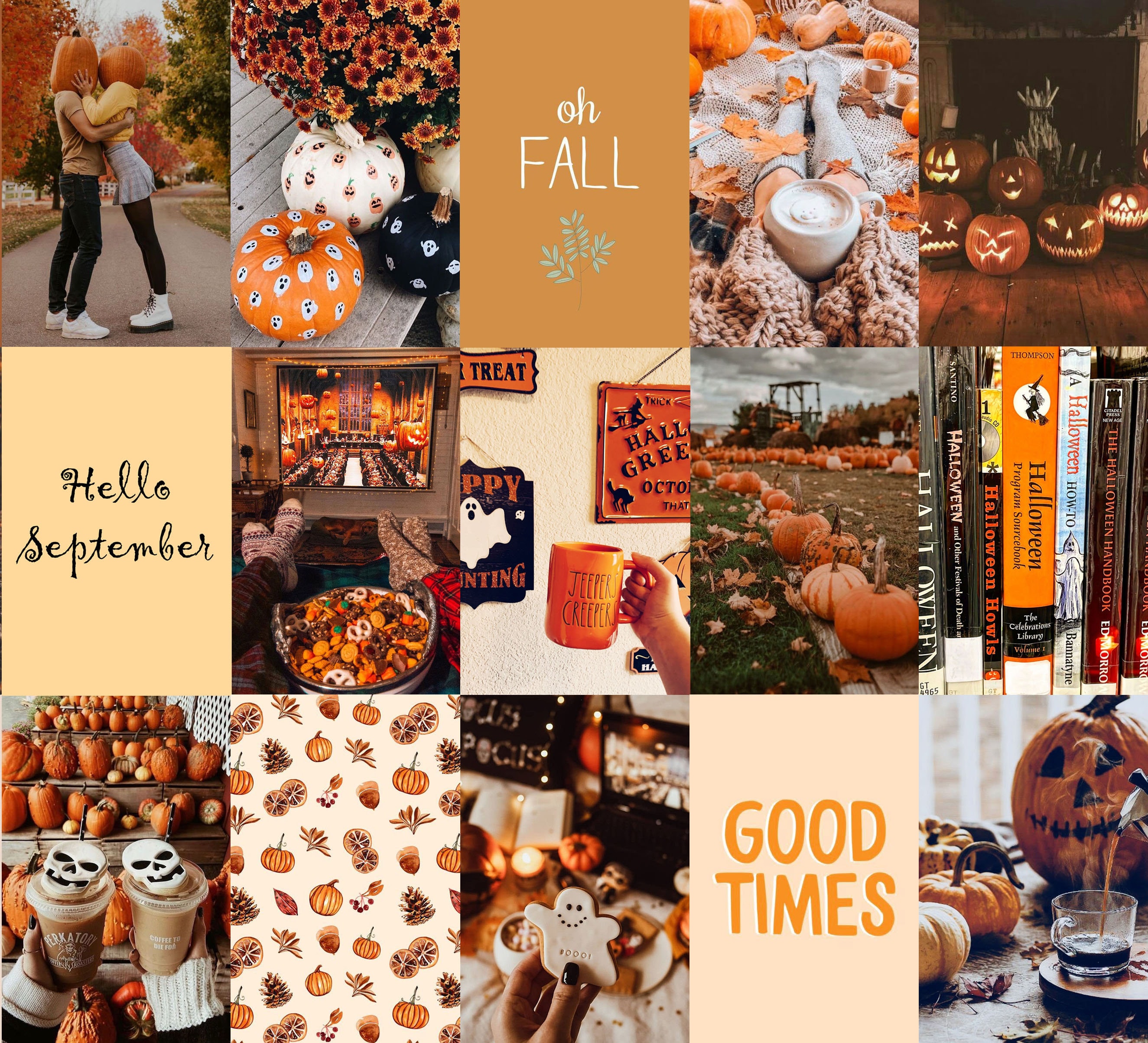The image is a detailed collage divided into three rows and five columns, featuring various autumn and Halloween-themed scenes. Each section of the collage is a square containing unique imagery paired with festive captions. 

- In the first row, the third column displays the text "Oh Fall." The last column of this row captures a group of jack-o'-lanterns.
- The second row's first column features the text "Hello September," while the last column reveals a collection of books about Halloween.
- In the third row, the fourth column has the phrase "Good Times."

Visually, the first row of the first column showcases two individuals wearing pumpkins on their heads, seemingly posed to kiss. The collage scenes prominently include pumpkins and related elements throughout, with one section featuring a faulty wallpaper, adding a rustic charm to the overall aesthetic.